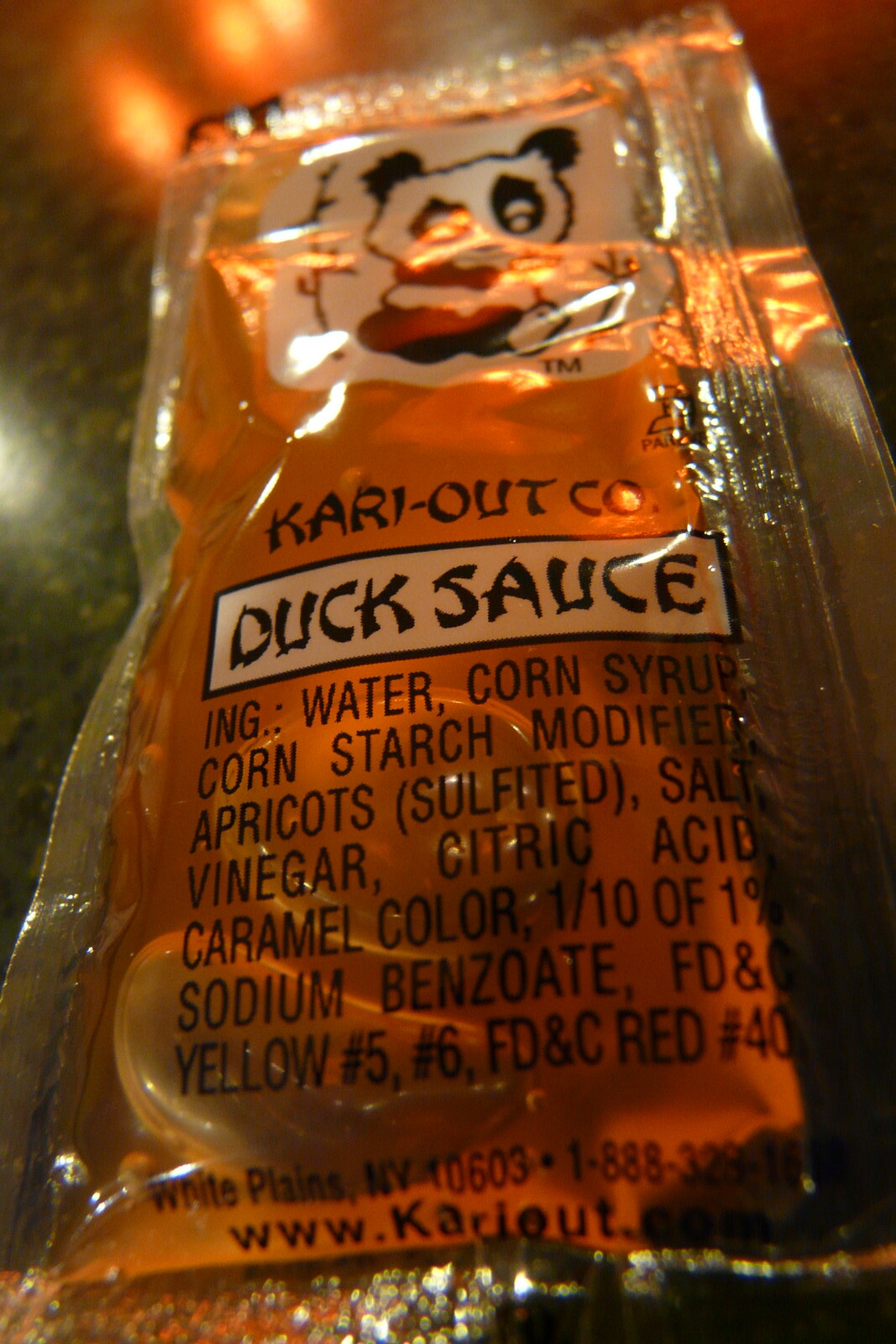This is an extremely detailed and close-up screenshot of a packet of duck sauce, positioned on a dark wood table in a dimly lit room. The image is slightly obscured by a glare, likely from dim lighting or a nearby candle, making some details harder to read. The sauce packet itself has a silver outline and features a small logo of a black-and-white panda bear at the top, which appears to be looking straight ahead. Directly beneath the panda bear, the packet reads "Carry Out Co." The words "duck sauce" are prominently displayed in a white horizontal rectangle with bold black lettering. Beneath this, there is a comprehensive list of ingredients, which includes water, corn syrup, modified cornstarch, apricots, salt, vinegar, citric acid, caramel color (1-10-19), sodium benzoate, and FD&C color additives Yellow No. 5, Yellow No. 6, and Red No. 40. The package also indicates the company's location as White Plains, New York, 10603, and provides a website and phone number, although both are somewhat indistinct due to the glare and the small size of the text. The sauce inside the packet is a yellow-golden color, and the overall appearance suggests a casual dining or takeout setting.